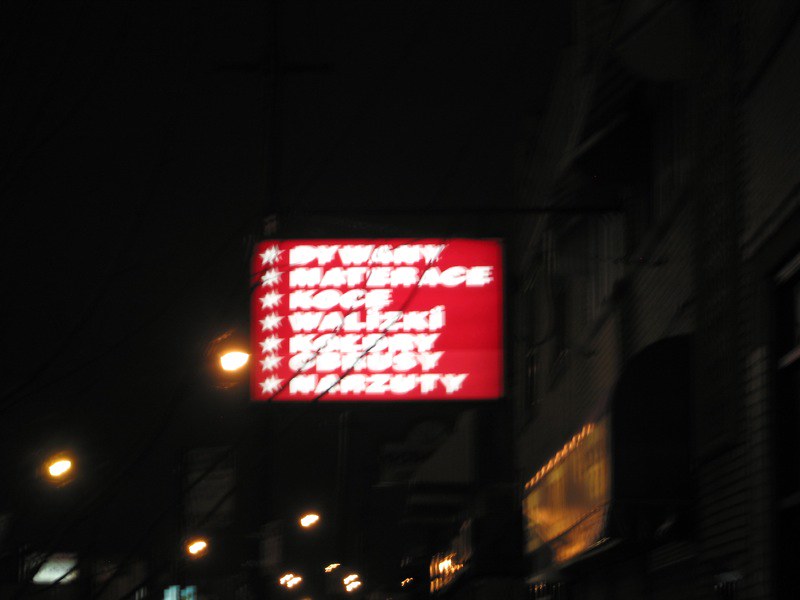The image showcases a nighttime scene captured outdoors. The sky appears completely black, and the overall picture is noticeably blurry. Prominent in the image are multiple circular, bright yellowish-white street lights, seemingly floating in the air as their supporting poles are not visible. A laminated red sign with white text stands out to the left side of the frame. The sign has 14 white stars aligned in pairs down its left side, with blurry white text next to each star pair that may indicate numbers or words. Part of the right side reveals barely discernible buildings dotted with orange lights and several blue lights at the bottom left. Within the darkened backdrop, there are a couple of black lines intersecting the scene, likely power lines, passing in front of the sign. The blurry inscription on the sign hints at the characters "K-O-C-E," but the rest remains indistinct.